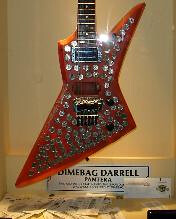A vibrant electric guitar, resembling a lightning bolt with its narrow, pointy form and adorned with bejeweled elements, takes center stage in this photograph. The guitar, predominantly orange with shimmering light reflections, boasts an array of silver embellishments across its face that could be coins or jewels. A cream-colored wall serves as the backdrop, with a sign beneath the guitar bearing the name "Dimebag Daryl" in black lettering, suggesting a tribute or display, possibly in a museum. Below the plaque, small items such as tickets or money are visible. The scene is illuminated from above, with fluorescent lighting casting a glow and enhancing the sparkle of the guitar’s intricate decorations. Only a portion of the fretboard is visible, extending upwards towards the top of the frame, emphasizing the guitar's striking design.